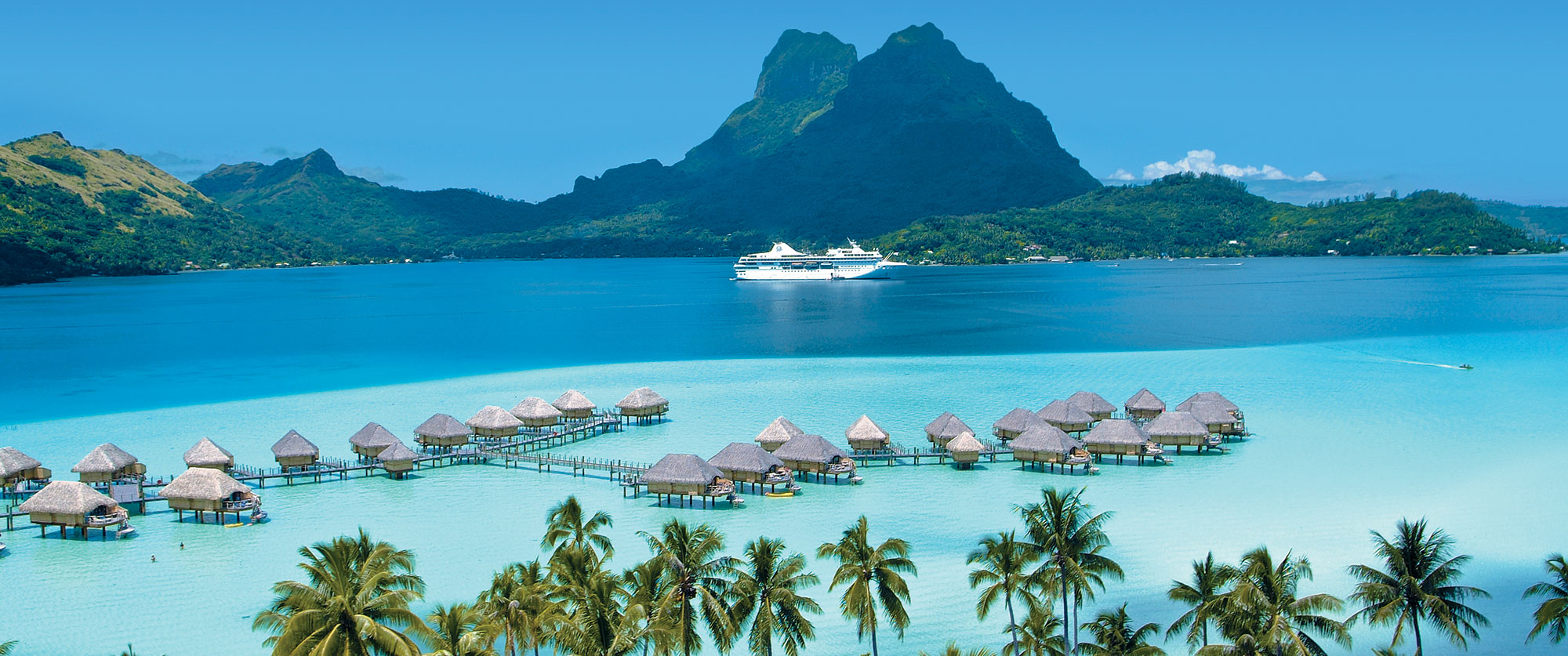This captivating image of a tropical paradise, ideal for a Bahama vacation ad, showcases a luxurious scene reminiscent of a Sandals resort. Rows of charming, yellow-brown huts with brown roofs extend over crystal-clear, light blue water, transitioning to a deeper, dark blue as it stretches towards the horizon. Palm trees with vibrant green tops frame the foreground, their trunks hidden from view. In the middle ground, a jet ski traces a dynamic path from the deeper blue waters to the shallows.

Dominating the background are lush, mountainous islands, their green peaks towering hundreds of feet above sea level, bathed in a barely clouded, vivid blue sky. A pristine white cruise ship with at least four visible levels glides gracefully past these verdant mountains, adding to the allure and adventure depicted in the scene. This detailed composition, featuring a perfect blend of serene waters, luxurious accommodations, and natural splendor, paints an irresistible picture of a dream Caribbean escape.